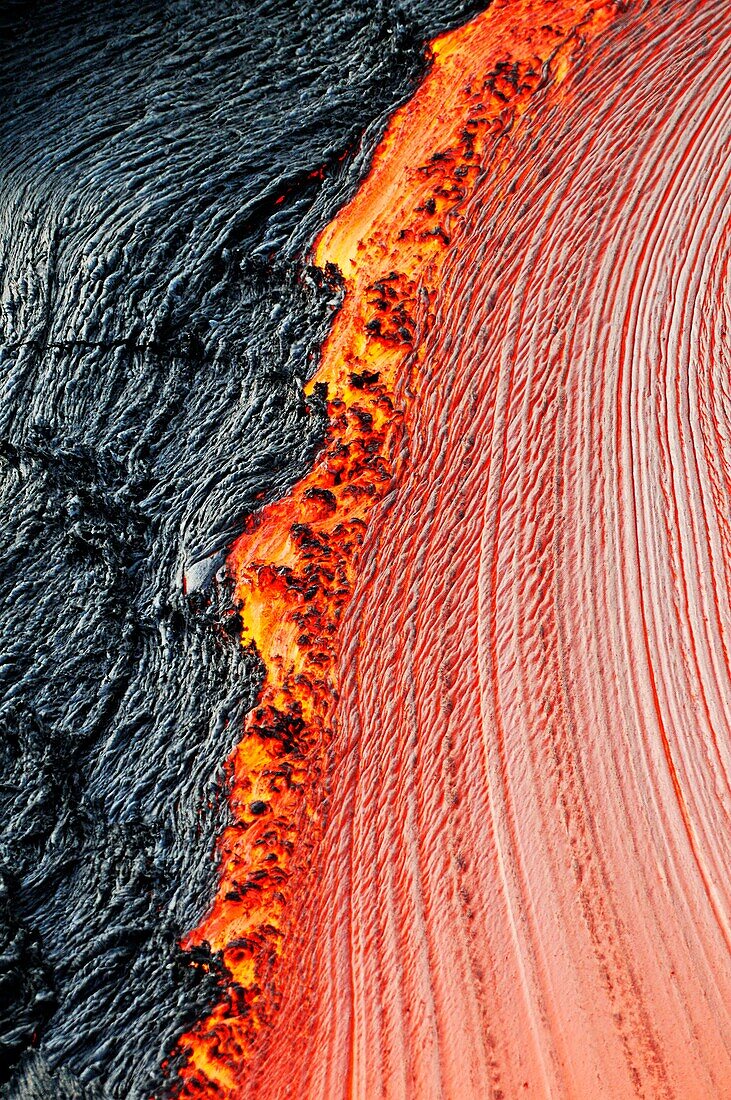The image depicts a highly detailed, close-up view of a volcanic lava flow in motion. The scene is dominated by a striking contrast between the intense, bright orange molten lava on the right side and the solid, dark black ash or cooled lava on the left. Flowing downwards in the center, the vivid orange lava, interspersed with hints of yellow and black, resembles a combed array as it cascades towards the bottom of the picture, creating a dynamic sense of movement. The right-hand side features peculiar formations akin to multiple roads, accentuating the intricate patterns of the flowing lava, whereas the left side remains a stark, unbroken expanse of dark material. The photograph contains no text, people, or other objects, focusing solely on the dramatic convergence and interaction between the hot, flowing lava and the cooler, solidified surface.